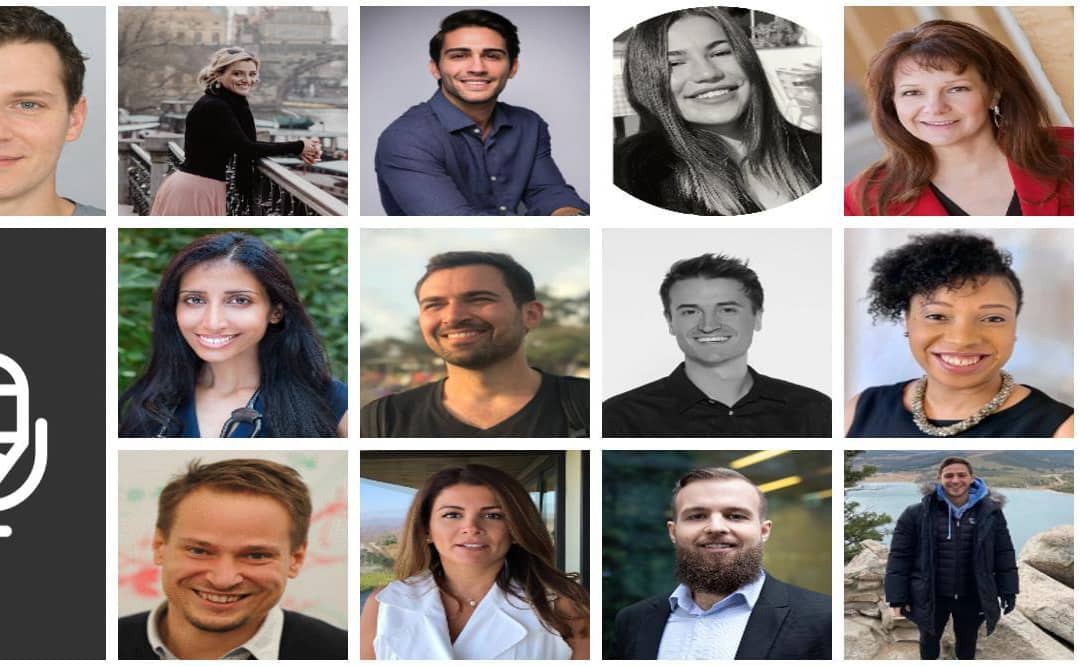This collage features various close-up images of people's faces and shoulders, organized into a grid. The top row consists of five individual portraits, while the row below contains four images, making up two rows of four images in total. On the lower right side, there's a man standing outdoors, wearing a coat. To the left side of the collage, beneath a partially cropped face, there is a longer rectangular section, suggesting a cut-off area within the image that includes what appears to be part of a microphone.